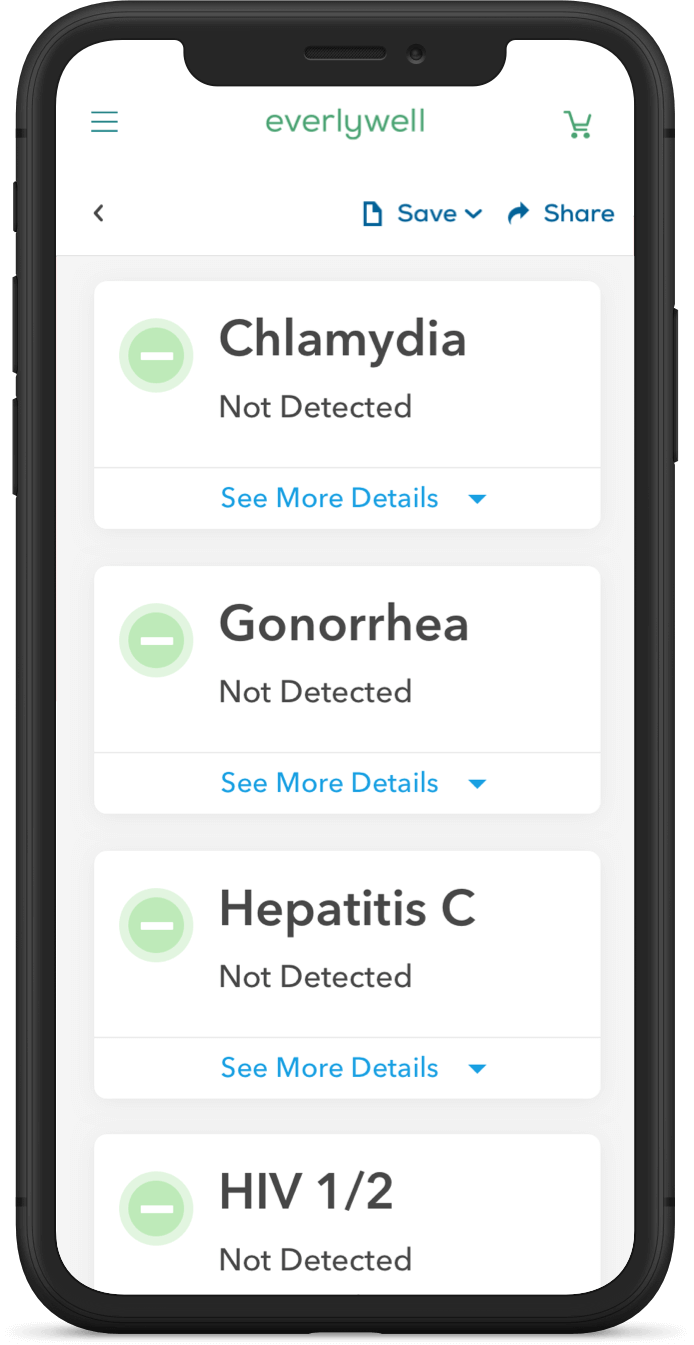A photograph captures the front view of a smartphone encased in a sleek black cover. The screen displays a white background with the title "Everly Well" prominently centered at the top. To the left of the title, a menu icon with three horizontal lines is visible, while a shopping cart icon appears on the right. Below this, on the right side, are three interactive elements: a save icon with a dropdown menu, a curved share arrow, and the word "Share."

The upper portion of the screen features four white rectangular boxes, each containing different health test results:

1. **Chlamydia: Not Detected** - Annotated with a light aqua-colored circle featuring a minus sign.
2. **Gonorrhea: Not Detected** - Also marked with an identical circle and minus sign.
3. **Hepatitis C: Not Detected** - Accompanied by the same circle with a minus sign.
4. **HIV 1/2: Not Detected** - With the usual circle containing a white minus sign.

Each results box includes a blue-text option at the bottom reading "See More Detail," paired with an arrow indicating a dropdown menu for further information. The image clearly documents the phone's screen and the specific test results displayed through the Everly Well application.